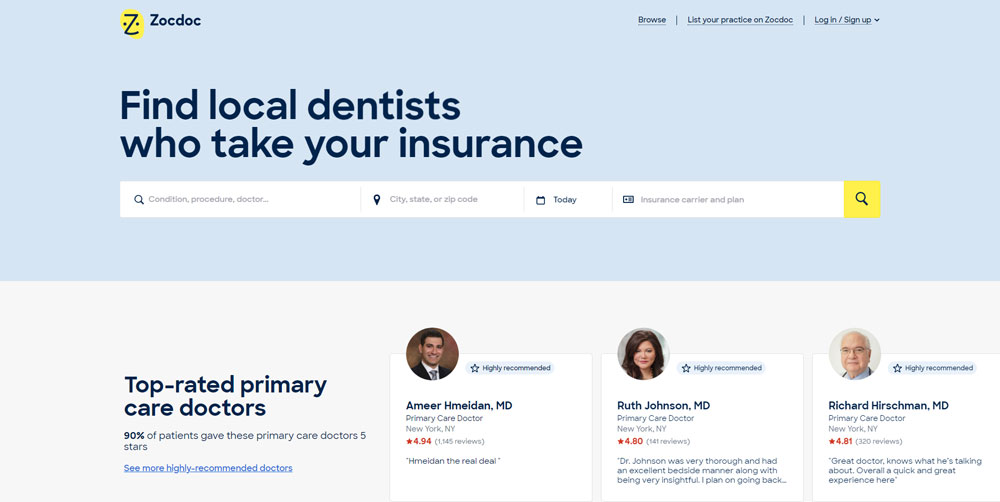This screenshot captures the homepage of the ZocDoc website. The top section features a light blue background. In the upper left corner, there is a yellow circle with a black 'Z' in it, flanked by two small black dots, representing the ZocDoc logo. Adjacent to the logo is the ZocDoc name in black font.

Directly beneath the logo, a bold statement in large font reads, "Find local dentists who take your insurance." Below this headline, there is a search field where visitors can input their condition, procedure, doctor, city, state, or zip code, along with their insurance carrier or plan. At the upper right side of the website, there are options to "Browse," "List Your Practice on ZocDoc," or "Log In / Sign Up."

Further down, beneath the blue section, there is a gray area. This area highlights top-rated primary care doctors with a statement in black font: "Top rated primary care doctors. 90% of patients gave these primary care doctors five stars. See more highly recommended doctors." 

To illustrate, three sample doctor profiles are displayed. The first profile features "Amir Hamidin, highly recommended primary care doctor, New York, New York." The second profile showcases "Ruth Johnson, MD, highly recommended primary care doctor, New York, New York." 

The structured layout and clear categories make it user-friendly for visitors seeking medical professionals covered by their insurance.